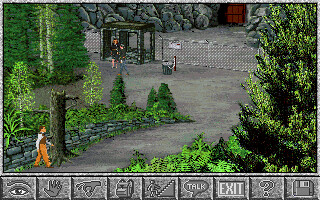A screenshot from an older point-and-click adventure video game is depicted here. The gray path winds between two rows of trees, leading the viewer's eye through the scene. On the right side, tall trees with lush green leaves dominate the image, providing a dense, forested backdrop. In contrast, the left side features smaller trees and varied foliage, adding depth and texture to the landscape. At the end of the path stands a silver-colored fence with a small booth beside it, adding an element of intrigue and potential narrative importance. Two figures are visible in the background, though their details are indistinct. In the foreground, toward the left, a character in striking orange pants and a white shirt stands prominently. Along the bottom of the screen, a user interface displays various icons: an eye, a hand, a hand gripping an item, a backpack, stairs, a speech bubble, an exit sign, a question mark, and a floppy disk, indicating different interactive options available to the player.